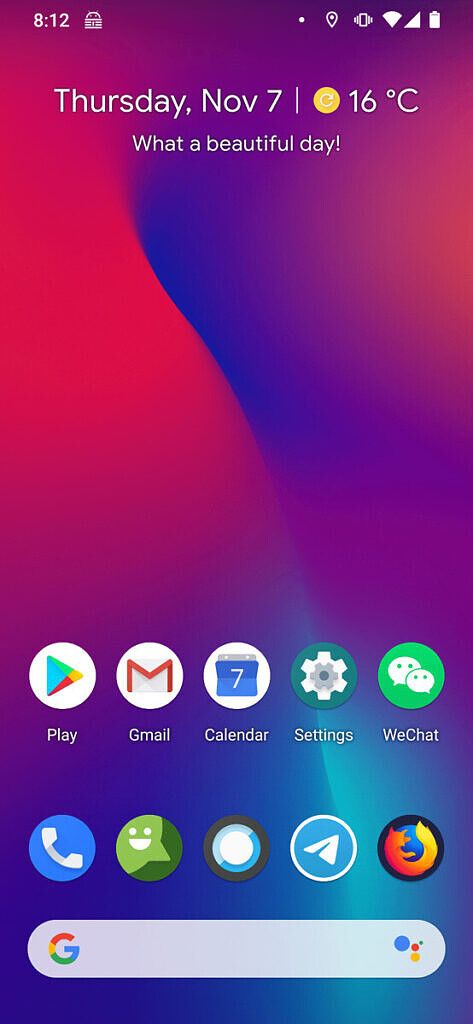This image showcases a detailed screenshot of a smartphone screen. The background features a captivating abstract pattern dominated by blues, pinks, and reds, with hints of white interspersed throughout. In the upper left corner, the time is displayed as 8:12. The upper right corner contains icons indicating Wi-Fi connectivity, cellular signal strength, and battery level.

Centered just below these icons, the date and weather information is presented: "Thursday, November 7th, 16 degrees Celsius. What a beautiful day!" This text adds a touch of personalization and context to the scene.

In the lower third of the screen, various app icons are neatly arranged. From left to right, there is the Google Play icon, followed by Gmail (depicted as a white envelope with a red 'M'), Calendar (a blue box displaying the number 7 in white), Settings, and WeChat. Below this row, additional app icons include the Phone app (a green circle with a smiley face) and the Mozilla Firefox icon on the far right. The combination of these elements provides a comprehensive visual representation of the phone's interface at a particular moment.